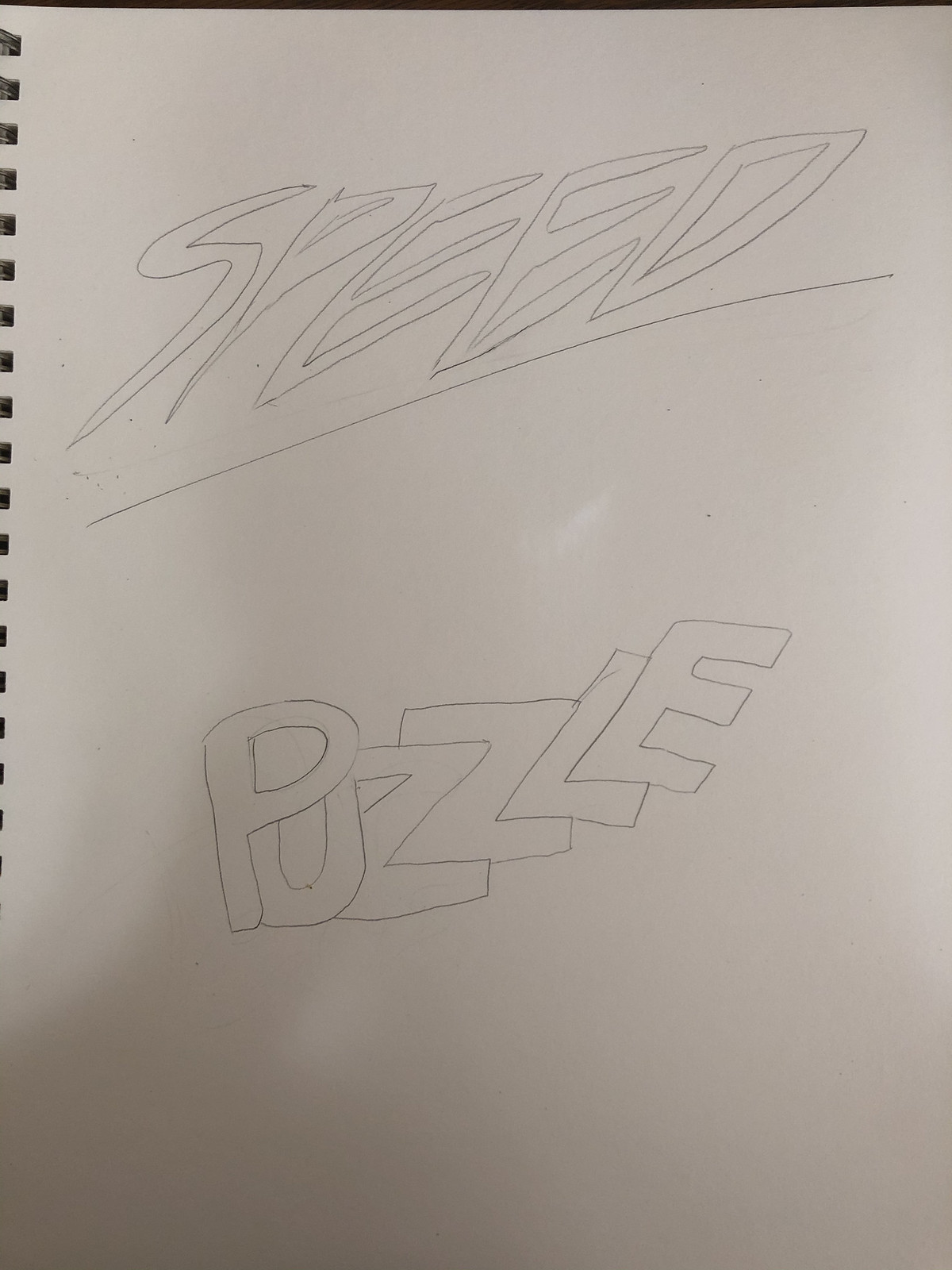This photo captures a partial view of a spiral notebook, revealing pages gridded with small, faint squares through which a black spiral coil weaves. The notebook is open, showing a pencil sketch on the left side of the page. The top edge of the paper is slightly visible, while the bottom edge remains out of the frame. Centered at the top of the page, the word "SPEED" is prominently written in angled bubble letters, crafted meticulously in pencil. An angled line is drawn just beneath this word, suggesting a dramatic emphasis or underline. Near the bottom of the visible page, the word "PUZZLE" appears in similarly stylized bubble letters, this time connected, adding a playful yet deliberate touch to the sketch. The strategic use of bubble letters and the careful arrangement of the words give the image a whimsical yet orderly aesthetic.